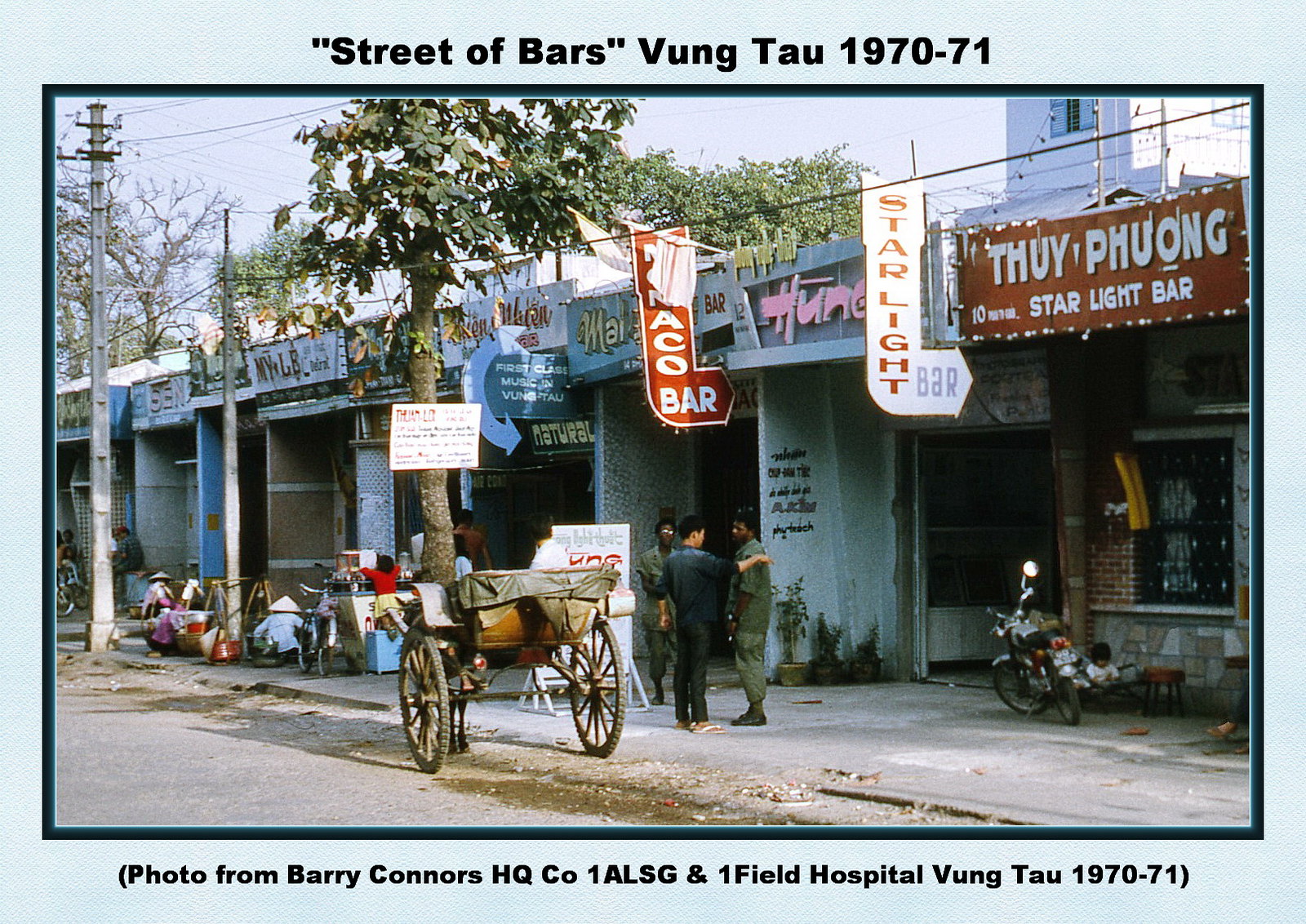The image, titled "Street of Bars, Vung Tau, 1970-71," features a vividly detailed street scene from Vietnam, captured by Barry Connors of HQ Co., 1ALSG, and 1 Field Hospital. The photograph, taken between 1970 and 1971, is bordered in light blue with the title text across the top and attribution along the bottom. The view shows a diagonal street perspective with a row of one-story storefronts, each marked with colorful signs in Vietnamese, signifying their function as bars. Notable names include the "Starlight Bar" and "Thuy Phuong."

The street is non-paved, with a somewhat uneven sidewalk. Visible in the scene are multiple people, including a man dressed in a green uniform and another in a blue shirt and black jeans. A motorbike is parked outside one of the bars, with a horse-drawn carriage seen nearby. Further details include a child seated on a brown stool, people donning iconic Vietnamese triangular straw hats, and lush green trees providing some shade. Overhead, power lines stretch against a mostly blue sky, adding to the scene's historical authenticity. The overall milieu is bustling yet slightly chaotic, capturing a vibrant slice of life from Vung Tau during the Vietnam War era.